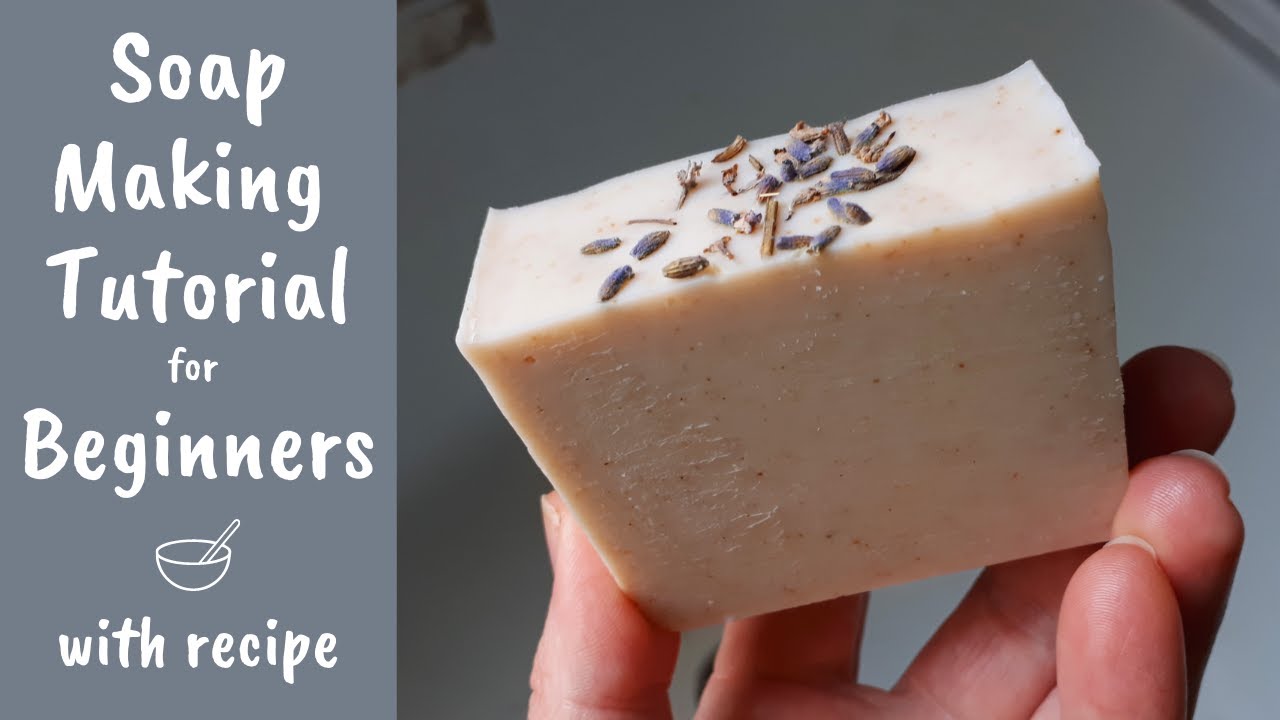This image appears to be a YouTube video thumbnail for a homemade tutorial titled "Soap Making Tutorial for Beginners with Recipe." The background is a grey or white color featuring a vertical grey rectangle on the left side with white text. The text includes the main title along with a simple drawing of a bowl containing a spoon or utensil. On the right side of the image, there is a person's left hand holding a bar of soap. This soap is cream-colored with visible seeds or herbs embedded on top, which gives it a somewhat purple hue. The overall composition suggests an instructional and inviting guide for beginners interested in soap making.